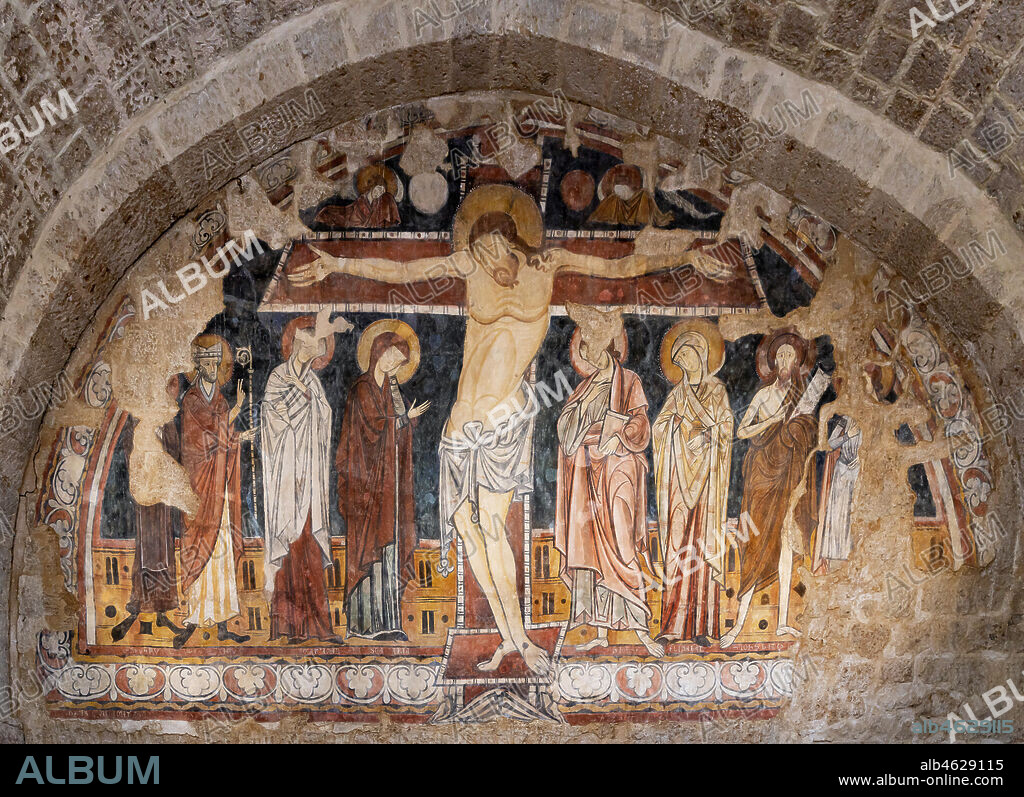In this image, a colored, vintage-style mural painting vividly depicts the crucifixion of Jesus Christ under a stone arch composed of layered bricks in various hues. The arch extends horizontally from the left middle side to the right middle side, disappearing out of the frame. At the center, Jesus hangs on a wooden cross, distinguished by his brown hair, golden halo, and minimal attire—a simple white cloth over his waist and upper legs. His arms are outstretched, displaying subtle marks at his hands and feet, indicative of the crucifixion.

Encircling Jesus, six figures—three on each side—appear, some adorned with golden halos, suggesting their religious significance as apostles or followers. The figures, both men and women, are attired in garments reminiscent of the Jerusalem period. 

Throughout the image, the word "album" repeatedly appears in white, slanting from the bottom left up towards the right. These inscriptions vary in boldness, with some faint and others more prominent, including one crossing Jesus's waist. A black border runs along the bottom of the image, featuring the word "album" in blue on the left corner. On the right side of this border, white text reads "ALB-4629115" followed by "www.album.com."